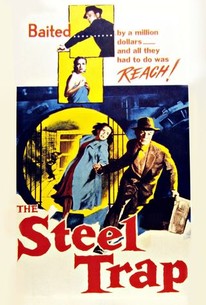This vintage movie poster for the 1952 Warner Brothers film "The Steel Trap" features a predominantly white background with artistic hand-drawn and colored illustrations. Dominating the top of the poster, a man in a blue coat and black fedora is running away, accompanied by a smaller image below of a woman holding a towel to her chest. The red text above them reads, "Baited by a million dollars and all they have to do is reach." In the center, the main illustration depicts the same man, now in a brown suit and brown fedora, holding onto the hand of a woman in a blue coat and red dress. The scene is set under a police searchlight with policemen visible in the background, suggesting a tense, dramatic moment. The bottom of the poster prominently displays the film's bold red title, "The Steel Trap." Additional smaller square illustrations within yellow rectangles are interspersed between the text at the top and the central image, adding to the poster's vintage charm.